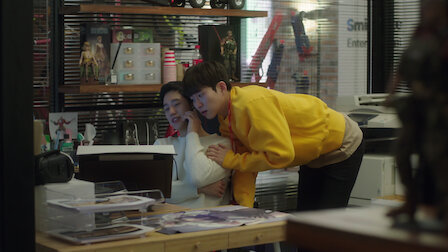This image captures an office scene with two young men, one seated and the other standing closely beside him. The setting is an office space adorned with various items and decorations. The seated man, dressed in a long-sleeve white sweater, is positioned at a desk that holds multiple objects, including trays for paper and other office supplies. He appears to be engaging with a computer screen or possibly a phone call, given his focused demeanor.

Standing behind him is another young man in a yellow long-sleeve sweater with black pants and possibly a brown shirt underneath. He leans in closely, his right hand resting gently on the seated man's forearm while their heads nearly touch, giving the impression that he is either listening to the phone call or looking at the same screen. The expressions and proximity suggest they are deeply engrossed in a shared activity or discussion.

The office environment is detailed with a variety of elements: a shelf on the left wall crammed with small knickknacks and figures, and glass panels that give a view into and out of the office, adding a sense of openness to the space. In the background, additional office equipment, including what may be a copier, further accentuates the business setting.